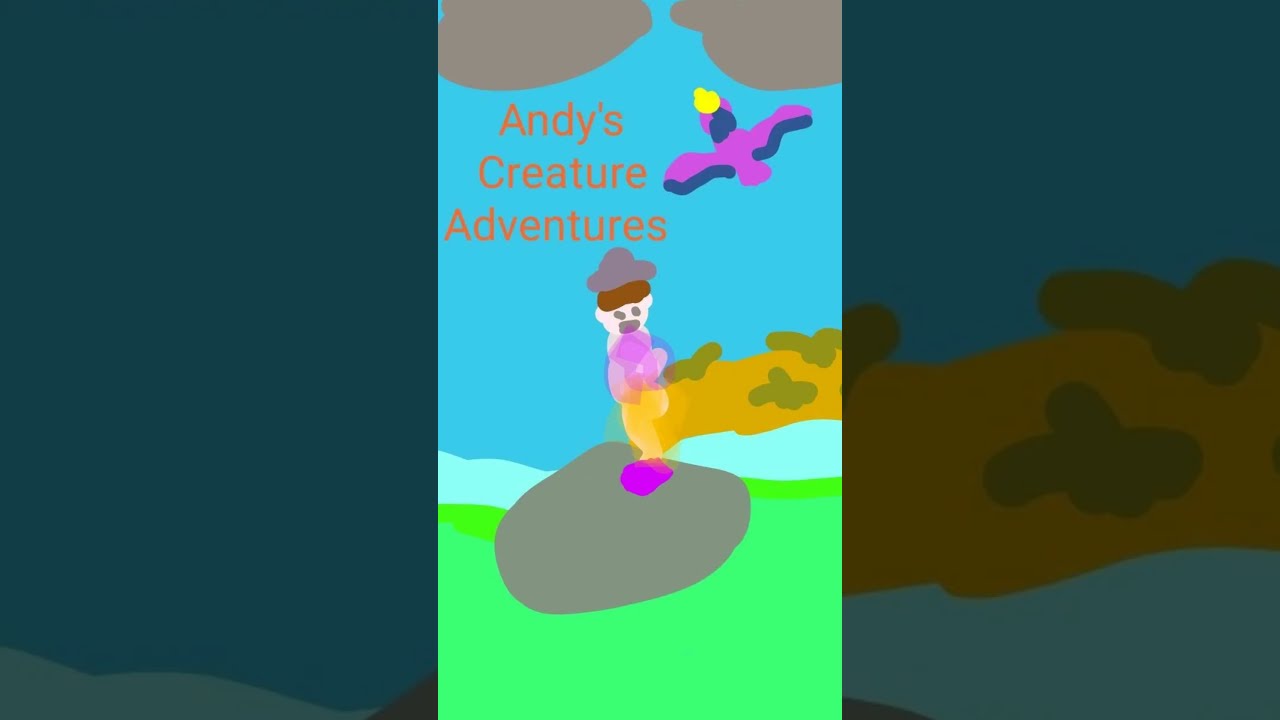This image appears to be a primitively drawn computer artwork, possibly created using Microsoft Paint. The vertical rectangle features a scene titled "Andy’s Creature Adventures," indicated by white text in the upper portion, spread across three lines. The backdrop is a solid blue sky, home to two grey clouds located in the upper corners, with the left one slightly larger than the right. A vibrant blue bird with a yellow beak and purple accents is seen soaring toward the clouds. Below this, a character, presumably Andy, stands centered on a grey rock. Andy is depicted as a white-skinned boy with brown hair, wearing a grey hat, a purple shirt, yellow pants, and mismatched purple shoes. The foreground is composed of light pastel green grass, with Andy's rock rooted on it. To the right of Andy, there lies a yellow shrub flecked with orange or green splotches, partially covering what seems to be a grey rock or terrain. The sides of the image showcase close-up details of the drawing, each section overlaid with a semi-transparent black layer, presenting a surreal, vignette-like effect.